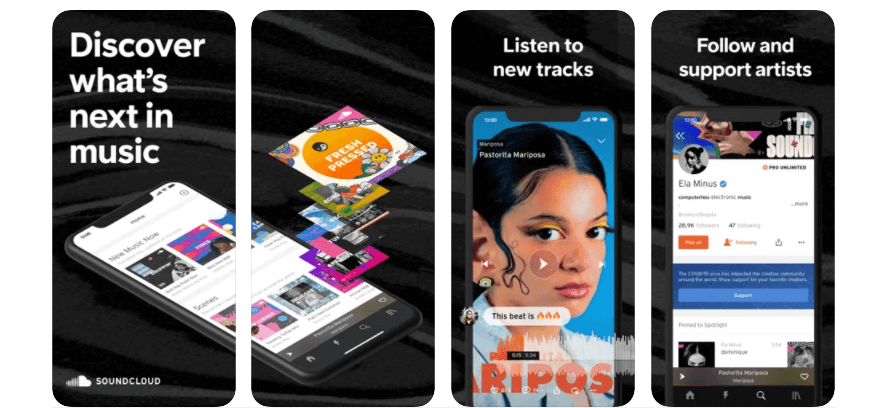This image consists of four panels resembling the shape of a smartphone screen, serving as an advertisement for SoundCloud. The panels have a uniform black background and are separated by a small gap of approximately one centimeter.

In the first panel, the SoundCloud logo and name are positioned at the bottom left. The top half of this panel features the text "Discover what's next in" alongside the illuminated half of a smartphone, indicating it is actively playing SoundCloud.

The second panel continues the image of the smartphone from the first panel, maintaining the black background. Displayed on the smartphone screen are album covers that appear to be dynamically emerging from the screen, progressively increasing in size. Among them, the largest album cover, titled "Fresh Pressed," stands out prominently.

The third panel contains the text "Listen to new tracks," accompanied by an image of an artist named Pastoria Mariposa, who is gazing at the viewer. A caption, "This beat is fire," further emphasizes the appeal of the content.

In the fourth and final panel, the phrase "Follow and support artists" is accompanied by a screenshot of Ella Minus's social media profile on SoundCloud, encouraging viewers to engage with and support their favorite artists through the platform.